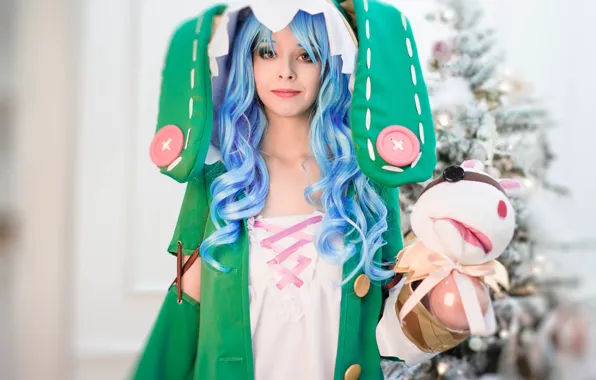In the photograph, a young white woman with long, wavy blue hair, appears to be cosplaying in a whimsical, festive outfit. She is wearing a light pink dress adorned with dark pink crisscross ribbons on the top, paired with a green coat that features large bronze buttons and a matching hat with large pink buttons resembling ears. Her blue hair and lipstick give her a striking appearance. In her arms, she holds a stuffed cow toy, which is nestled into what looks like a woven cone. The background, although blurry, reveals a white Christmas tree covered in artificial snow, suggesting a holiday setting. The scene captures her standing and posing in front of this backdrop, giving off a fun, Christmassy vibe reminiscent of a fantastical Christmas mermaid.